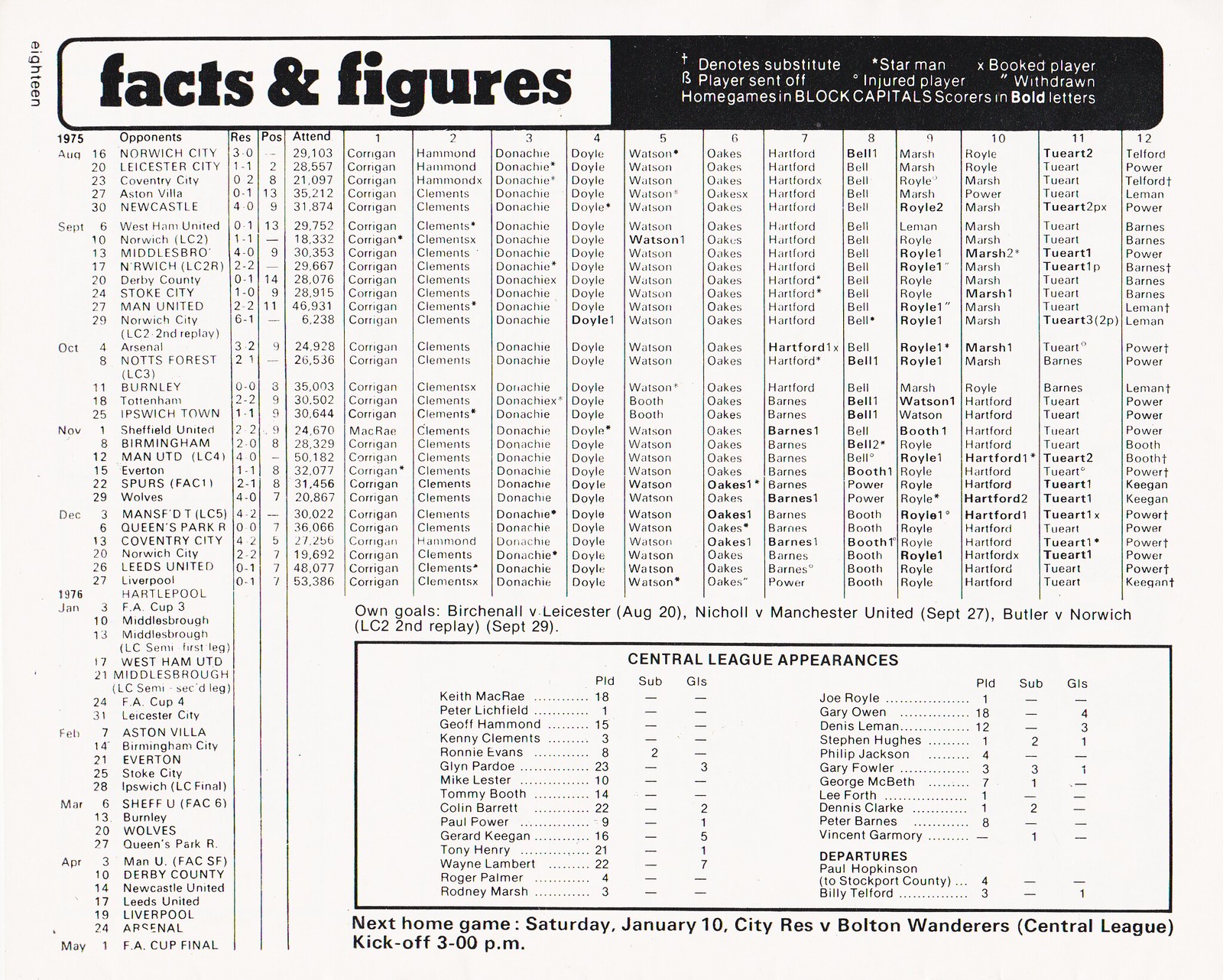The image displays a detailed scorecard or datasheet for a soccer game from 1975, resembling those found in newspapers before the internet era. The background is white with predominantly black text, featuring rows and columns filled with data. At the top, the heading "Facts and Figures" is prominently displayed, setting the tone for the comprehensive information below. This datasheet includes details such as the months from August to May, opponents, points, attendance, and locations of games. There are also player statistics, indicated by various symbols for substitutes, star players, booked players, players sent off, injured players, and withdrawn players. Home games are highlighted in block capitals, and scores are in bold letters. At the bottom right, it reads "Central League Appearances," listing multiple players and their details. Additionally, it mentions the next home game on Saturday, January 10th at 3:00 PM, featuring a match between City Reds and Bolton Wanderers in the Central League. The overall appearance and style strongly evoke a newspaper or magazine article dedicated to soccer team statistics and player information from that era.